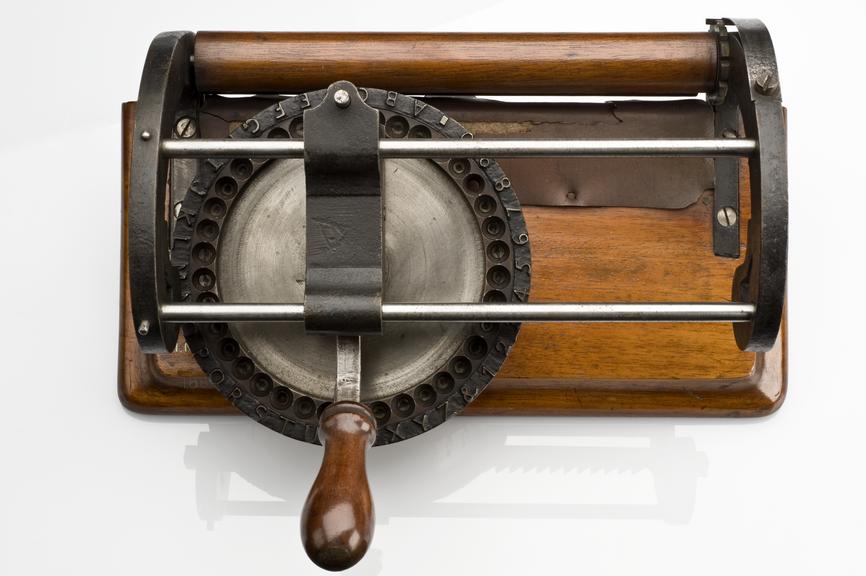This horizontally aligned rectangular image showcases an old-fashioned mechanical device. The centerpiece of the image is a medium to dark brown wooden base, horizontally aligned, set against a light gray or white background. The device features thin metal rods running across the wooden base—one at the bottom and one near the middle. Central to the apparatus is a circular tool with a dark wooden handle extending towards the viewer. The circular tool has a metal center, silver in color, surrounded by black metal that likely contains letters or numbers arranged around its edge. This circular component appears to be a wheel with small punch holes, possibly used to print or stamp. Overall, it’s an intriguing antique piece, combining elements of wood and metal, with the handle suggesting it might be operated by cranking to activate its mechanism.